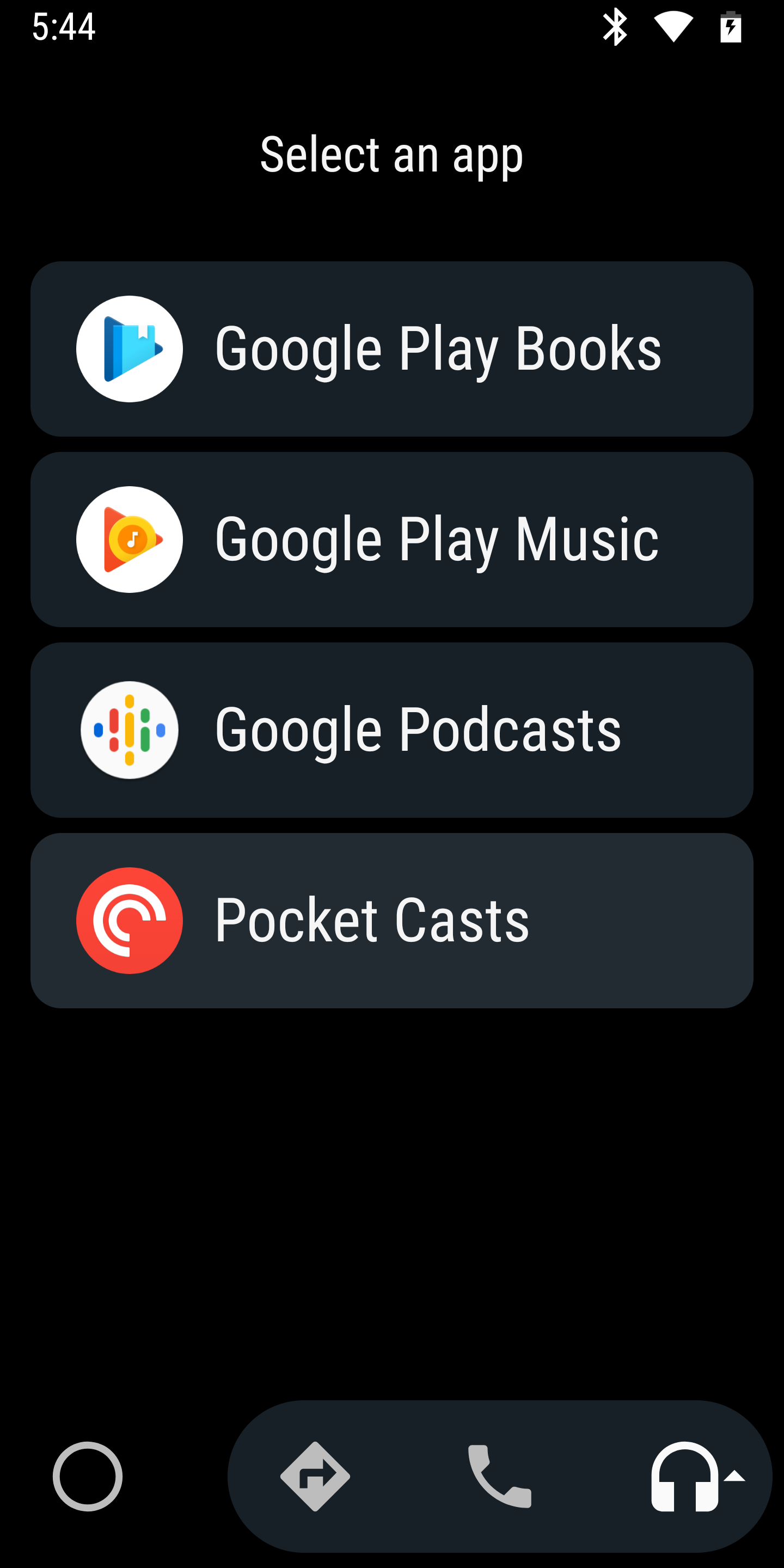This image is a screenshot of an app selector interface on a smartphone, captured in night mode. At the top left of the screen, the time is displayed as 5:44, confirming the device's status as a smartphone. On the top right, there is a battery icon, which appears to be slightly over half full and is also charging, indicated by a black lightning bolt within the battery symbol.

In the upper section of the screenshot, "Select an App" is displayed in white text. Below this instruction, a list of apps is visible including "Google Play Books," "Google Play Music," "Google Podcasts," and "Pocket Casts." This suggests the interface is designed for choosing an app specific to reading or listening to content such as audiobooks or podcasts.

At the bottom of the screenshot, there are several icons. The rightmost icon, which is highlighted in white, depicts headphones, indicating it is currently selected. To its left, there is an icon representing a phone, followed by an icon resembling a street sign with a 'back' arrow, possibly for navigation, and finally an empty circle icon located at the bottom left.

Overall, the user appears to be navigating an app selection menu, likely for managing multimedia content.